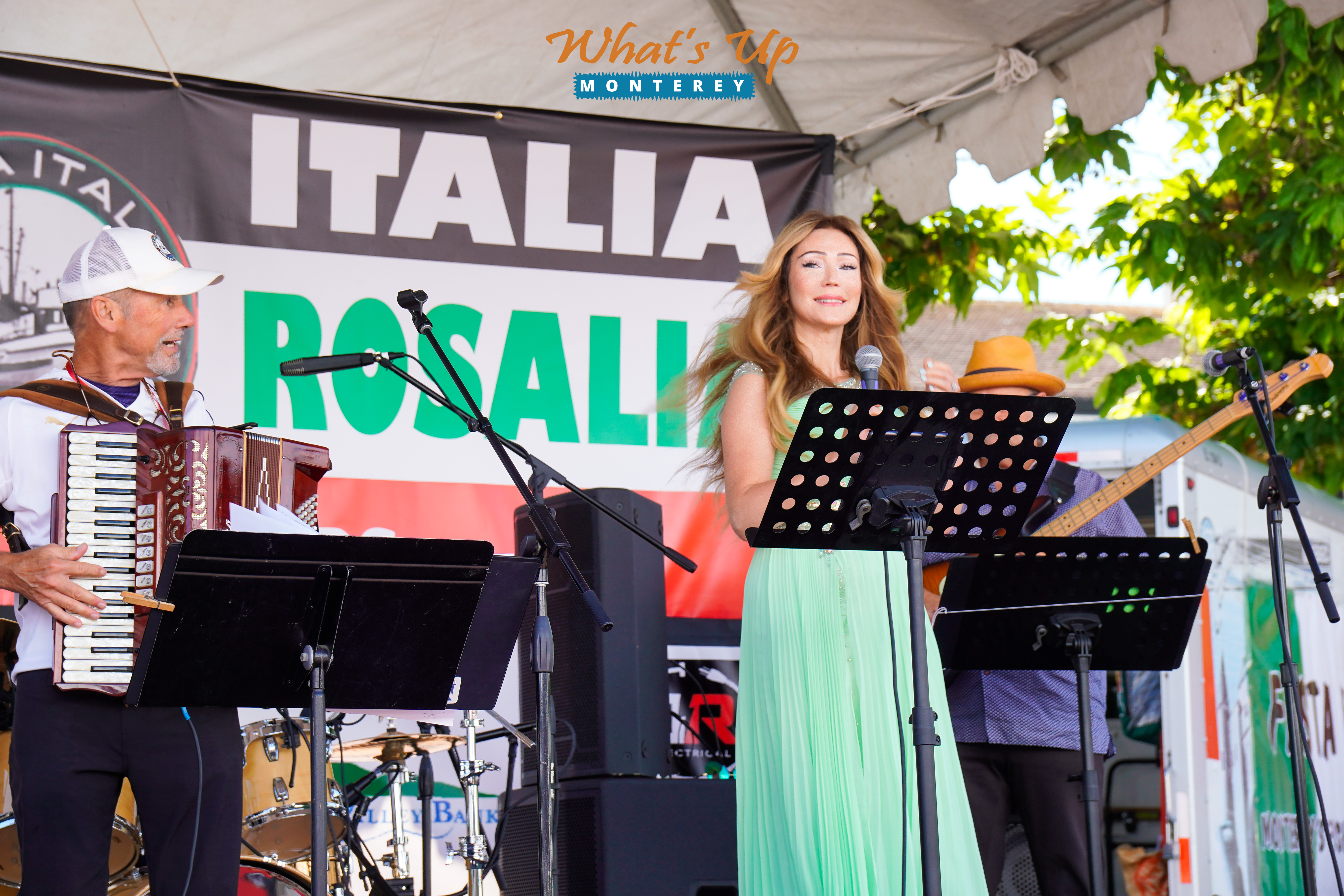The image captures a vibrant moment of a musical performance under a light gray fabric tent. At the top center of the horizontally aligned, rectangular picture, "What's Up" is written in medium brown text, followed by "MONTEREY" in bold white letters against a blue background. Center stage is a woman with long, flowing, light brown hair that cascades over her shoulders and slightly billows behind her. She wears a light green dress and holds a microphone, seemingly smiling as she looks toward the camera. 

To her left stands a man, possibly in his 40s, donning a white baseball cap, white shirt, and black pants. He plays a keytar, the keyboard’s black and white keys clearly visible as he holds it against his chest. In front of him is a black rectangular music stand. Behind the woman, another man is partially visible, identifiable by his orange hat, blue polka dot shirt, and dark pants. He holds a guitar while standing behind his own distinctive music stand with vented circles.

The backdrop features a large banner with the text "Italia Rosalia" partially obscured by the performers. This energetic scene conveys the dynamic interaction and engagement between the musicians as they perform together on stage.